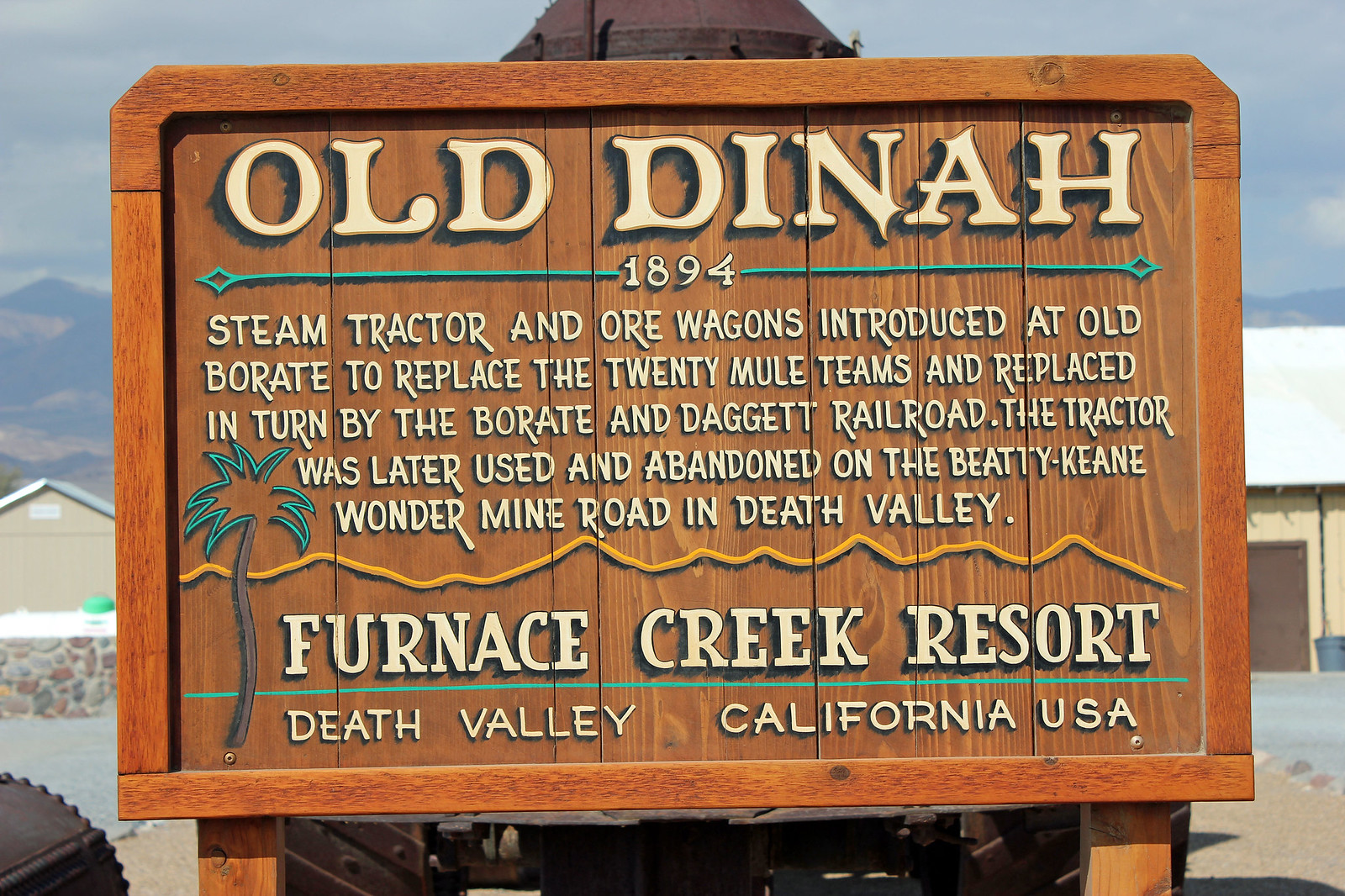This is a horizontally aligned rectangular photograph featuring a large wooden informational sign attached to two wooden posts. The sign is made of an attractive reddish wood and prominently occupies the foreground. In the background, a gray sky and mountainous outlines form a scenic backdrop, while on the ground, there appears to be gravel and a brown building with a white roof visible to the right. 

The sign itself is framed in wood and has a brown background. Across the top, large white all-caps letters read "Old Dinah." Below this, a teal-green horizontal line with arrows pointing left and right frames the year "1894" in its center. The body of the sign provides historical context: "Steam tractor and ore wagons introduced at Old Borate to replace the 20 Mule Teams and replaced in turn by the Borate and Daggett Railroad. The tractor was later used and abandoned on the Beatty Keene Wonder Mine Road in Death Valley." This description is left-aligned.

A light brown zigzag line separates this historical text from the information at the bottom, which reads in large yellow letters, "Furnace Creek Resort," followed by a teal horizontal line with "Death Valley, California, USA" in smaller white letters below. Additionally, on the lower left corner of the sign, a brown tree trunk with teal green palm tree leaves adds a decorative touch. This sign offers a well-rounded historical explanation of the feature visitors are observing.